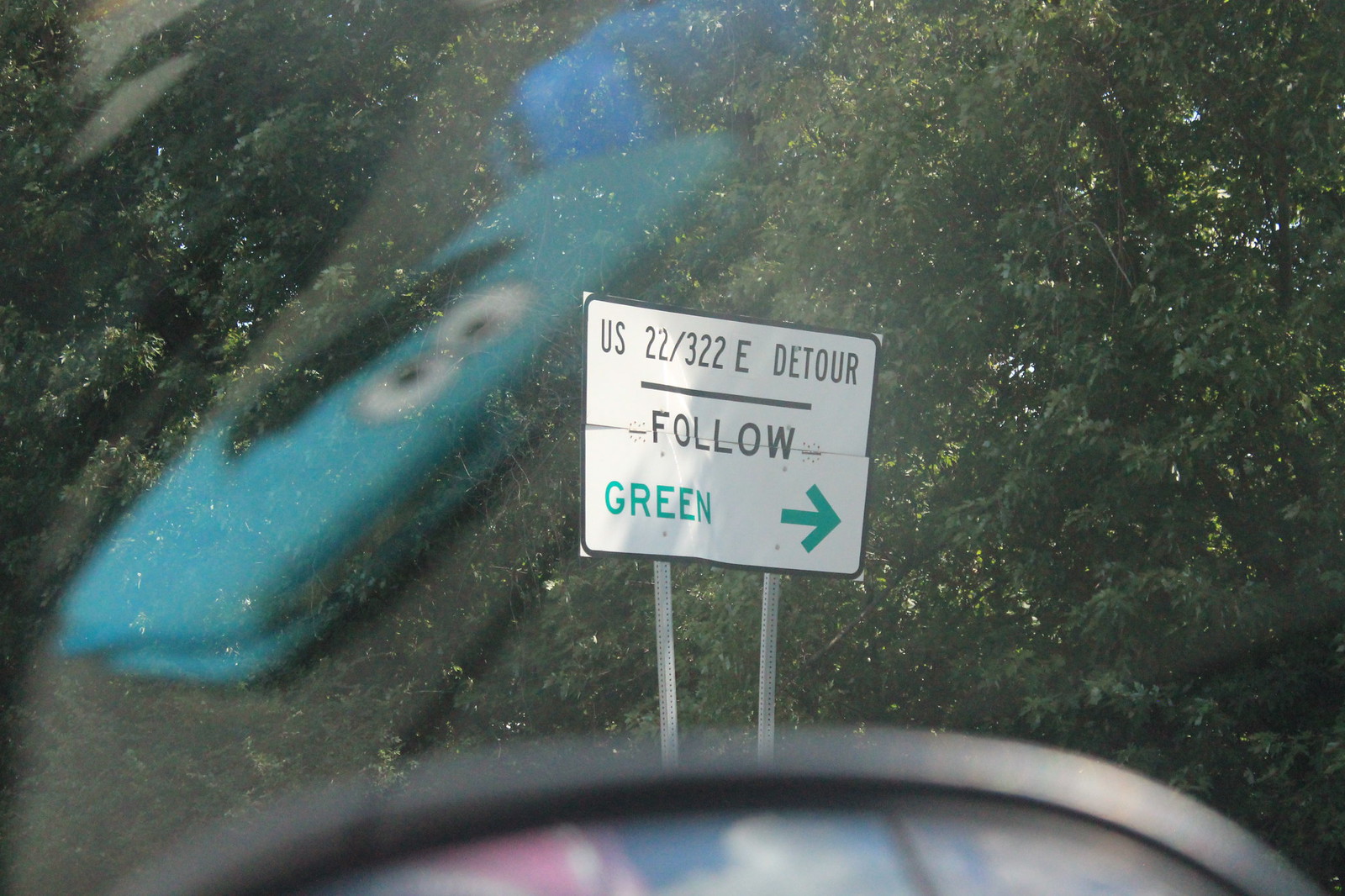A surreal and likely AI-generated image combines multiple disparate elements into a single, enigmatic visual. The background is composed of densely packed, green-gray trees resembling a forest. On the left side of the image, a gray solid background appears with a light blue flattened bag, complete with a black handle and two large, white eyes with black pupils. Above this peculiar bag is another small blue object. Below these elements is a section suggesting the interior of a vehicle, featuring a rounded black component. Emerging from this section is a street sign displaying "U.S. 22/322 East Detour" in black text, with a subsequent line reading "follow." The sign also features a green word "green" alongside a green arrow pointing to the right. This collage of seemingly unrelated objects creates a puzzling and intriguing composition.